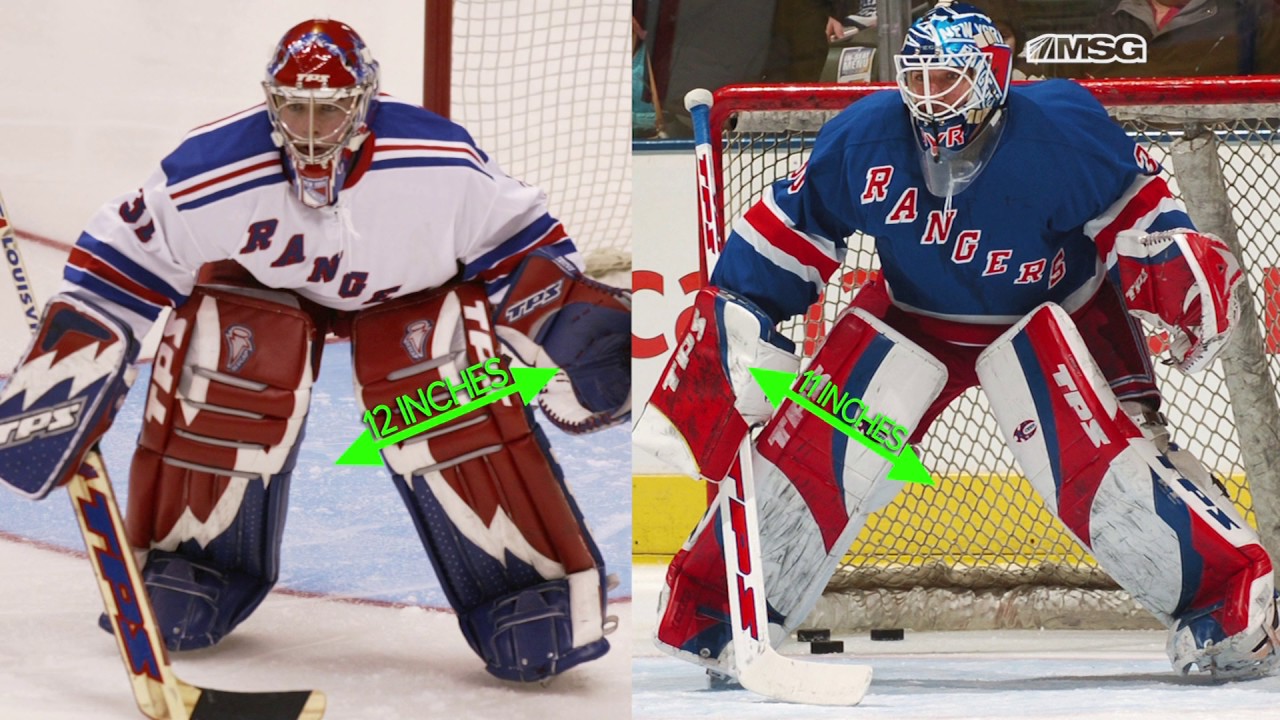The image depicts two NHL goalies from the New York Rangers side by side on the ice, potentially highlighting different uniform styles or the same goalie in home and away colors. The goalie on the left is dressed in a white jersey with blue and red accents, typical of a home uniform. The setup includes blue and red stripes and possibly the number 31, though not clearly visible. On the right, the goalie dons a blue jersey with red and white details, likely the away uniform, also showcasing "Rangers" scripted in red across the chest. Both goalies are shown in a crouching, guarding position with a red net visible behind the right-side image. A notable element is the focus on their leg pads; green text with arrows points to their width, indicating 12 inches on the left and 11 inches on the right. This detail might be under scrutiny for rule compliance or equipment comparison. The ice surface is evident beneath both players, enhancing the authenticity of the game scene.